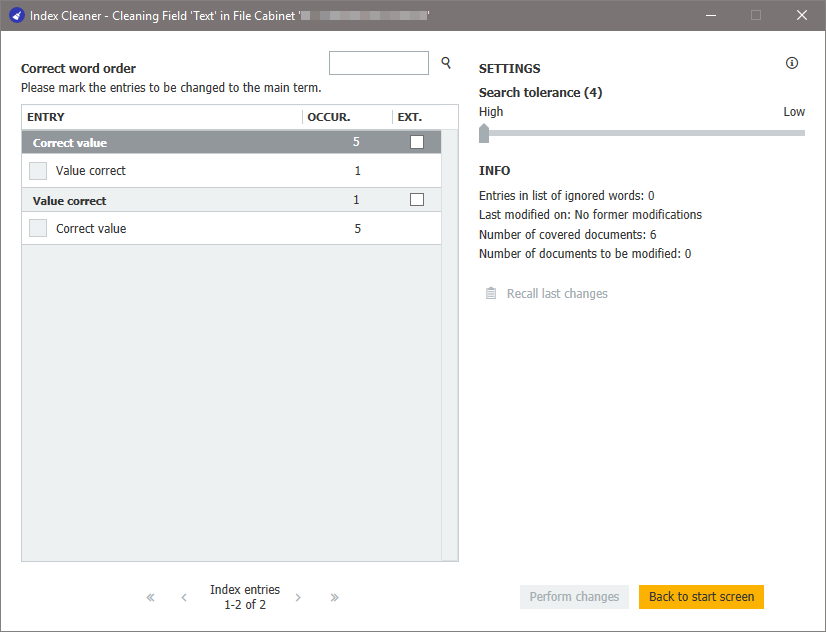The image depicts a desktop or laptop screen showcasing the "Index Cleaner" program. In the upper left-hand corner, a gray bar extends horizontally, featuring the text "Index Cleaner: Cleaning Field Text in File Cabinet" in white font. Adjacent to this text, also in the upper left, is a white paintbrush icon set against a small blue circle, likely serving as the Index Cleaner's logo.

Below the gray bar, on the left-hand side, the program displays options for "Correct Word Order." Directly underneath this, instructions prompt users to "Please mark the entries to be changed to the main term." 

Moving to the middle upper area of the screen, there is a blank search bar allowing users to input search queries. Below "Correct Word Order," there are two distinct categories labeled "Correct Value." 

Each category includes a checkbox labeled "Value Correct," followed by another instance of "Correct Value." Users can select the "Correct Value" checkbox to apply their desired changes within the Index Cleaner program.

At the bottom of the screen, on the right-hand side, a yellow bar provides two actions: "Back to Start Screen" or "Perform Changes," enabling users to either return to the main menu or execute the specified cleaning tasks.